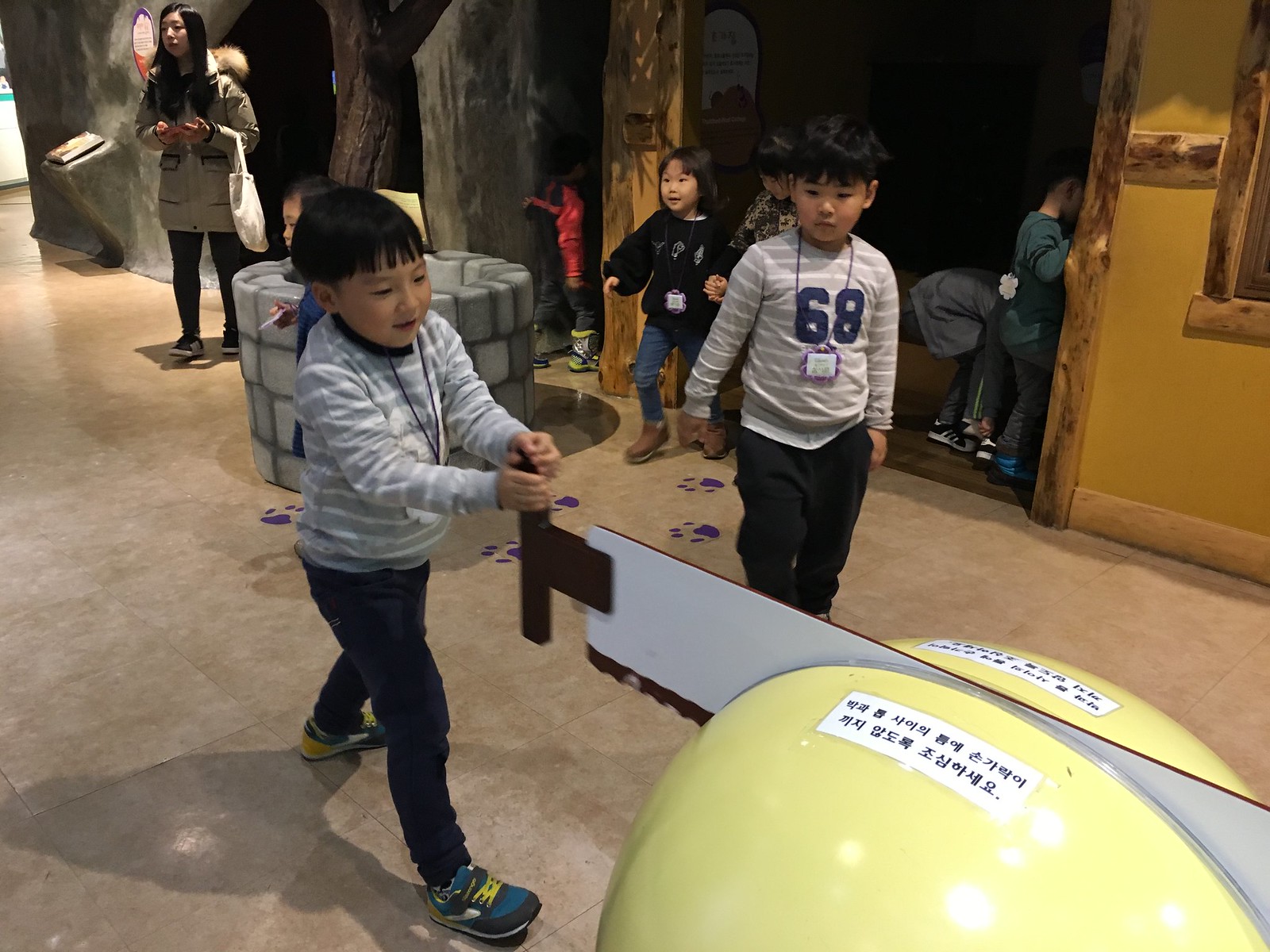The photograph captures a lively scene of children exploring a bustling children's museum. At the forefront, two boys, approximately five to eight years old, are deeply engaged in an interactive exhibit. Both boys wear dark pants with gray and white striped shirts, one of which features the number 68 on the front. They are equipped with lanyards, indicating participation in the museum's activities. One boy is engrossed in "sawing" a yellow metallic sphere in half using a white saw with a brown handle. The yellow sphere is adorned with Chinese characters on a white placard.

In the background, the museum reveals more playful settings: a makeshift house or hut painted in light brown with wooden sides, housing children who appear to be of Asian descent, aged three to five years old. Visible behind the saw exhibit are other children playing near a pretend well made of stones on the tiled floor. 

A distant adult woman, clad in a light brown jacket and holding a purse by her wrist, oversees the activities. She, too, appears to be of Asian descent with long black hair and looks towards the left side of the room. The environment is completed by a mock cave structure at the back, featuring light gray fake rocks, adding to the immersive, imaginative setting of the children's museum.